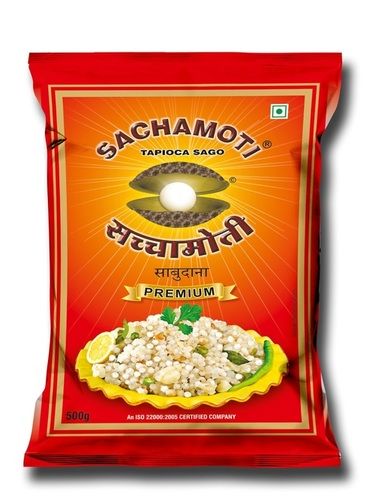The image depicts a vertically-oriented bag of Tapioca Sago pearls from the brand Satchimati. The bag itself is a striking reddish-orange color, with a prominent centrally placed rectangle displaying the brand's logo and a picture of the product. At the top of the bag, the brand name "Satchimati" is written in bold, brown capital letters, followed by "Tapioca Sago" in smaller black letters. The logo features an image of a large clam or oyster shell with a gleaming white pearl at its center, illuminated by rays of sunlight. There is a gold banner indicating that this is a premium product.

Below the logo, in a foreign language, additional information is provided. Further down, there is an image of a prepared dish showcasing the Tapioca Sago pearls, garnished with a lemon slice and some green cilantro leaves. The lower left-hand corner of the bag displays "500G" in black text, indicating the weight of the contents. Lastly, a smaller green and white square with a green circle in the middle appears in the upper right-hand corner, possibly indicating certification or another quality mark. Overall, the design and details of the bag suggest it is a high-quality product with emphasis on its premium nature and appealing presentation.